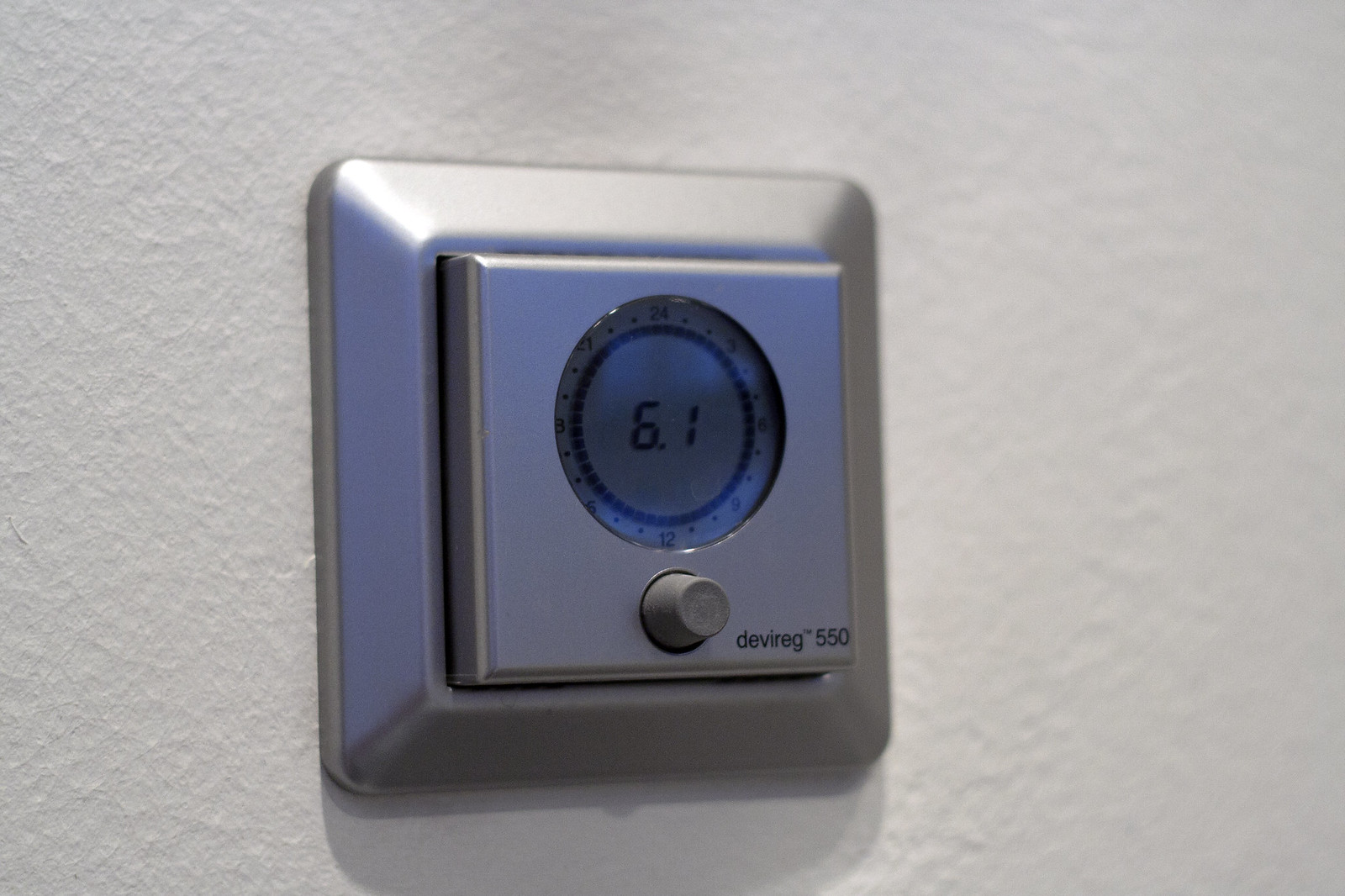The image showcases an electronic thermostat device affixed to a white, rough-textured plaster wall. The thermostat is a DEVIREG 550 model, as indicated by the label in the lower right corner. The device features a sophisticated design with a square silver base plate and a silver thermostat device seamlessly integrated into it. The main interface of the thermostat includes a 24-hour LCD clock face, with '24' at the top and '12' at the bottom, hinting at its European origin. The display shows the temperature "6.1," likely denoting degrees Celsius. Below this is a control knob fashioned from a darker gray plastic, contrasting with the brushed stainless steel of the overall unit. The clock face's LCD display has a neutral background with dark segments, and the temperature is displayed using a two-digit 7-segment format.